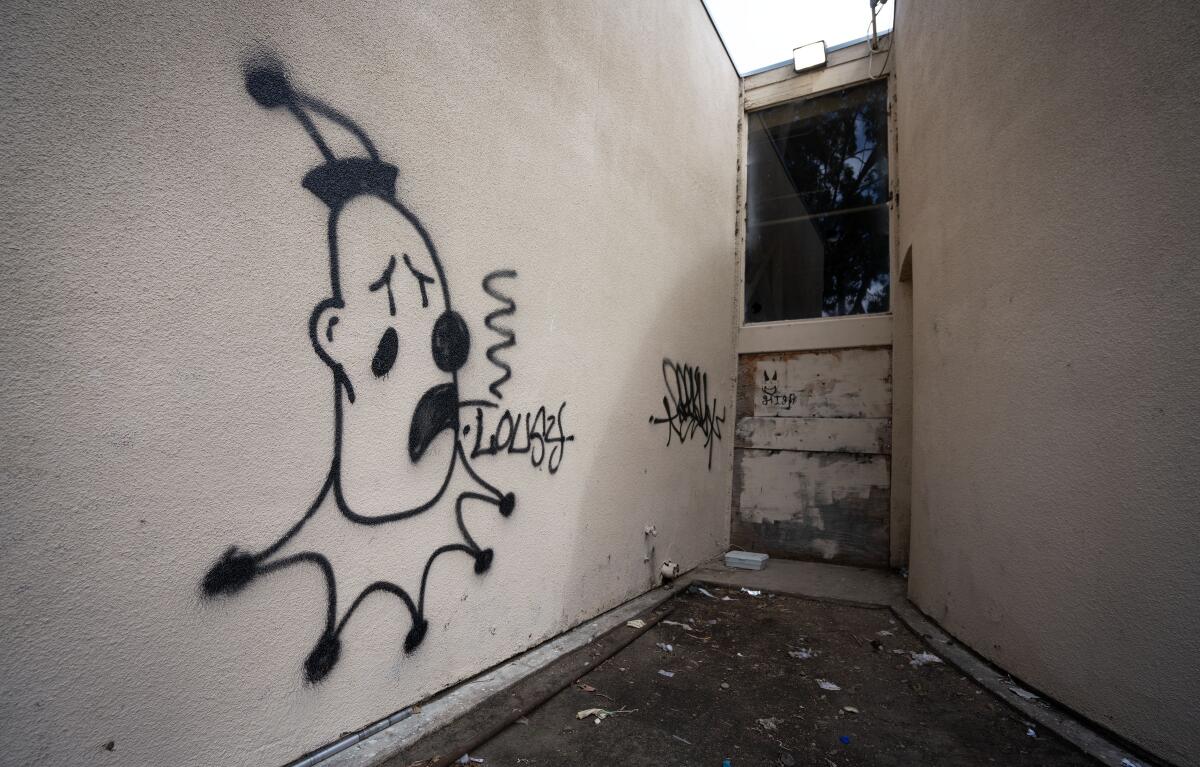The image depicts a scene that combines elements of decay and art, capturing a poignant street tableau. Set against a grey, possibly stucco wall, the graffiti portrays a sad clown with distinct black attire, characterized by a frilly costume around the neck and a pointed hat. The clown, who appears to be frowning, is depicted smoking, with visible swirls of smoke adding to the melancholic atmosphere. The graffiti is prominently featured near an entranceway that shows signs of wear and neglect, such as debris on the concrete floor and a boarded-up doorway with broken glass above it. The word "lousy" is scrawled near the clown's image, reinforcing the overall dour theme. The scene appears to be outdoors, perhaps in an alley or an industrial backyard, lending a gritty, nighttime feel to the composition.